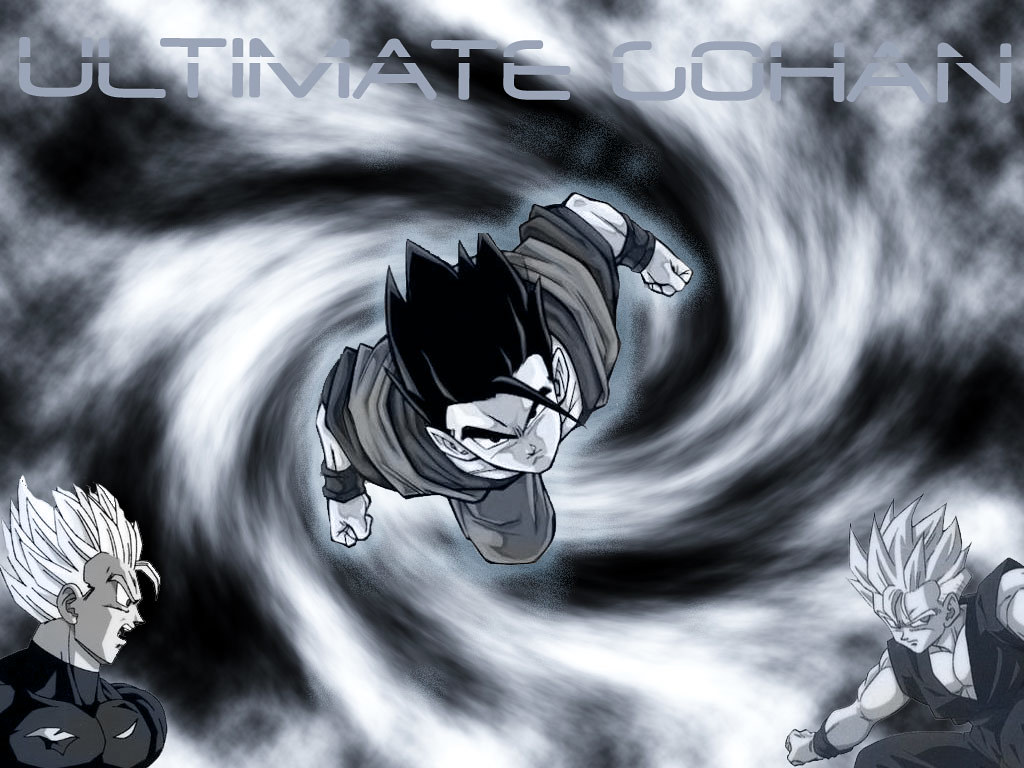The black-and-white image resembles the cover of a comic book or a screen capture from a cartoon, featuring characters in an anime style. Dominating the background is a swirling tornado effect. At the top, in bold, somewhat hard-to-read letters, it says "Ultimate Gohan." The central focus is a muscular young boy with black spiky hair, his fists clenched tightly, and a stern expression marked by dark eyebrows. He appears to be emerging from the tornado, almost as if flying. Positioned in the left and right bottom corners are two muscular males with spiky white hair and similar combat-ready postures, each with clenched fists and determined, angry looks on their faces.